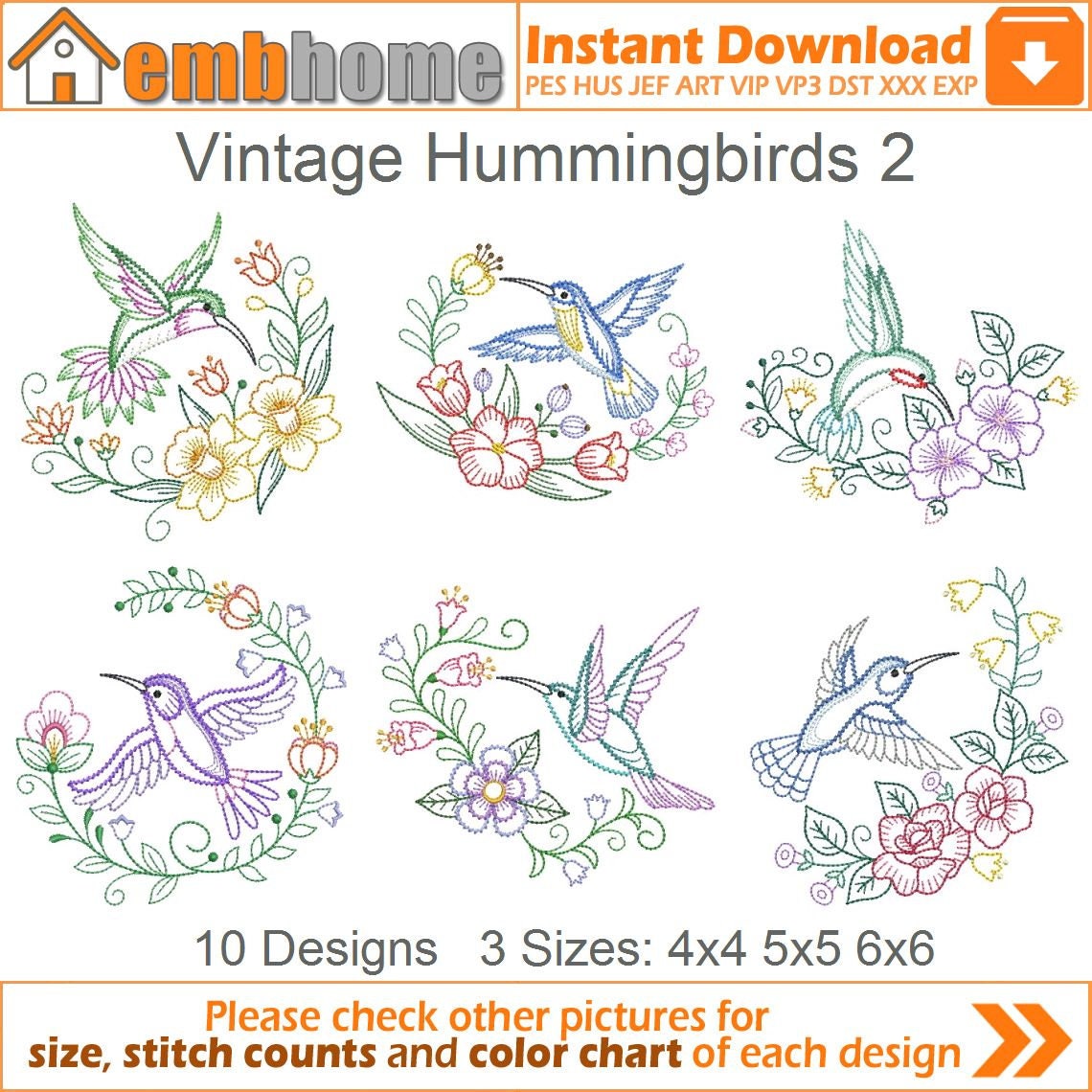The image showcases an embroidery pattern advertisement titled "EMB Home Instant Download Vintage Hummingbirds 2." The top of the image features a house icon with the words "EMB Home" and "Instant Download." Highlighted text specifies there are ten unique hummingbird designs, available in three sizes: 4x4, 5x5, and 6x6 inches. Each design prominently features a single hummingbird surrounded by a semicircle of various flowers. The hummingbirds and flowers vary in color and species, providing a diverse palette.

The detailed designs include:
1. A green hummingbird with purple accents on its wings and breast, surrounded by yellow daffodils and orange tulip-like flowers.
2. A blue hummingbird with a yellow breast amidst red, yellow, and pink flowers.
3. A green hummingbird with red cheeks, encircled by purple and yellow flowers.
4. A purple hummingbird framed by white flowers with pink and yellow details.
5. A green hummingbird with purple wings and tail, complemented by red and purple flowers with yellow trim.
6. A dark blue hummingbird with gray trim, hovering near red and yellow flowers.

At the bottom of the image, it advises viewers to "please check other pictures for size, stitch count, and color chart of each design," and includes two orange arrows pointing to the right. The background of the image is white, providing a clear view of each vibrant design.